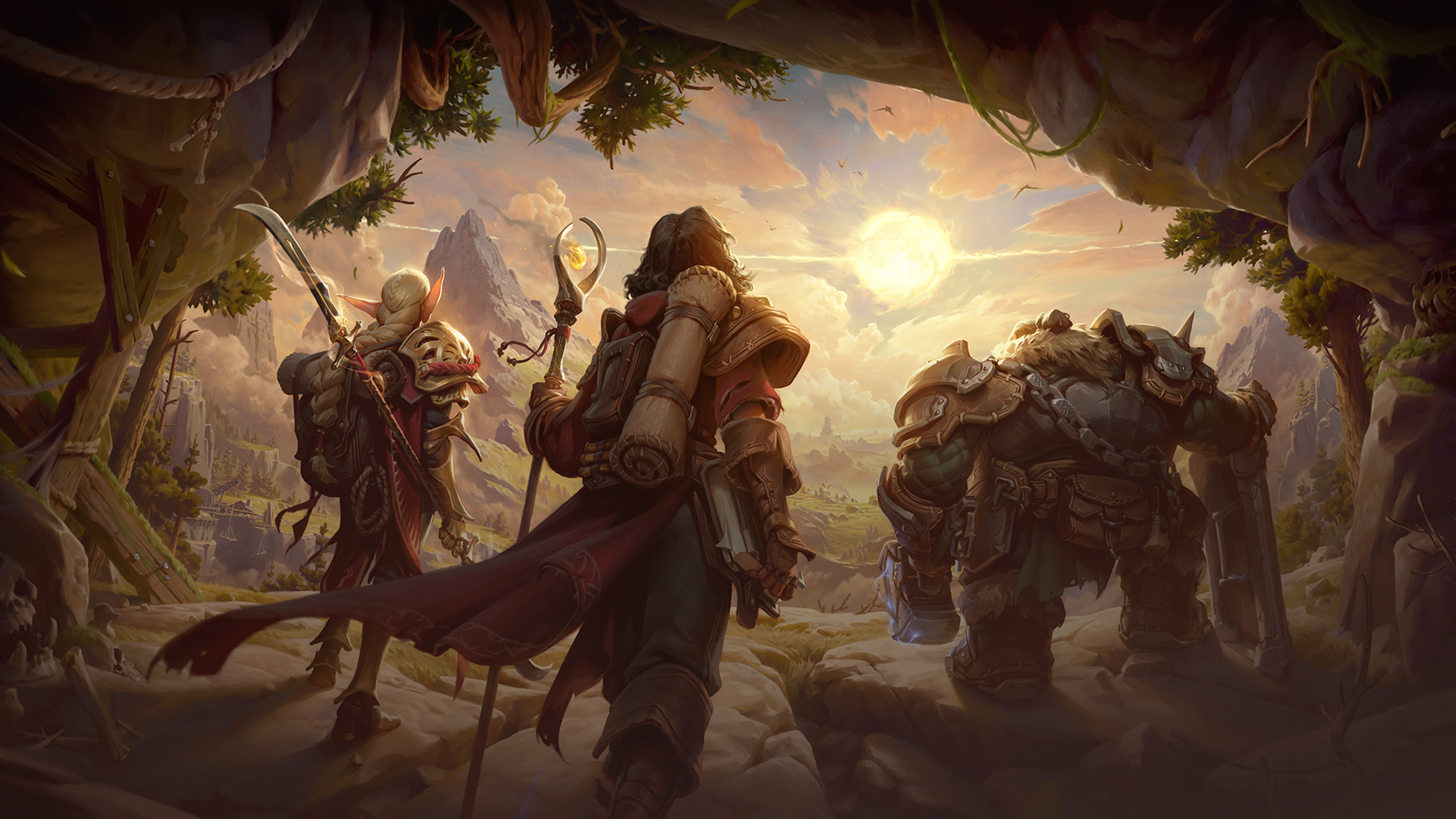In the fantasy painting, an epic adventure scene unfolds within a grey stone cavern, framing three distinct characters who stand at its mouth. The image centers on a glowing yellow sun, nestled among orange and white clouds in a blue sky, casting an ethereal light over the rugged landscape. To the left of the sun, a sharp grey mountain rises majestically.

In the foreground, towards the left, a blonde-haired elf with long, pointy ears stands poised. This elf carries a sword on its back with a long brown handle and a silver, curved blade that ascends to the top left. The central figure, draped in a red cloak, wears leather shoulder pads and gloves. This character, with long black hair, holds a staff topped with a twisted silver design in their left hand and bears a beige sleeping roll attached to a backpack.

On the right, a muscular, green-skinned creature commands attention. With a metal chain slung across its back, it grips a rectangular metal and wooden shield in its right hand, resting it against the ground. In its left hand, a broad metal hammer, crackling with blue electricity, points downwards.

The three adventurers stand united, gazing outward at the luminous sun, as if on the brink of an unknown quest. The cavernous surroundings, strewn with rocks and framed by the distant sunlit landscape, evoke a palpable sense of adventure and discovery.